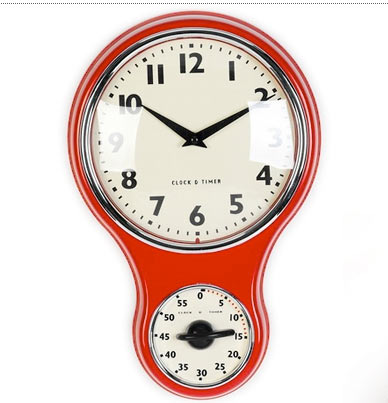The image features a wall clock set against a white background. The clock is housed in a shiny red frame that is a large circle at the top and curves down to encompass a smaller circle below. The main clock face is white with clear black Arabic numerals and black hands. The clock face is covered by a glass dome, which reflects light, giving it a slightly unreal perfection. The clock bears the label "Clock D Timer." Below the main clock, the frame extends to hold a second smaller gauge. This gauge also has a white face with black numbers and a black hand, marked from 0 to 60, currently indicating 13. This lower gauge resembles a timer or barometer and is similarly encased in the red frame, maintaining a unified and elegant appearance.